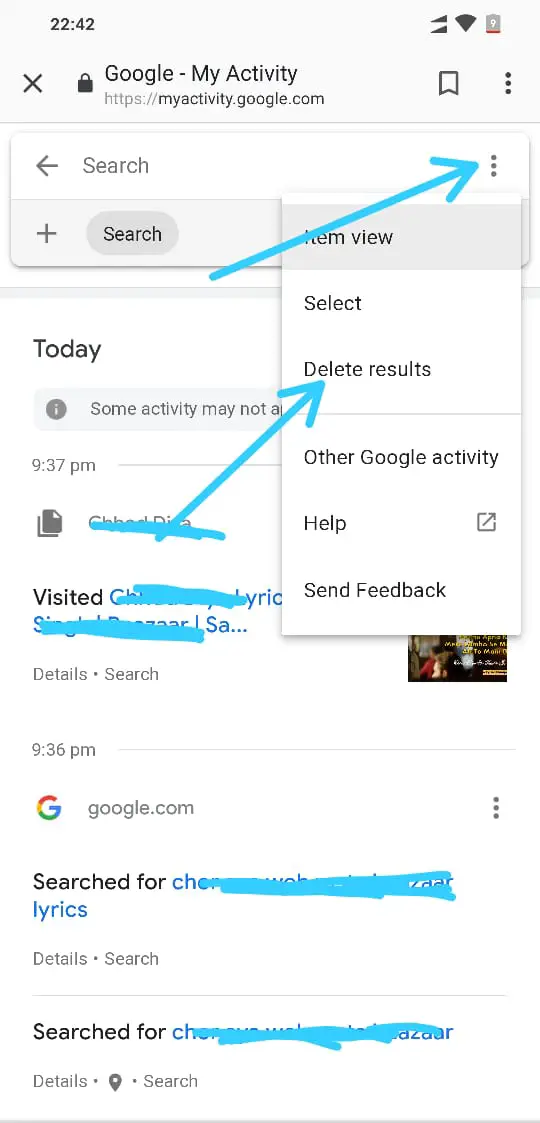The image is a screenshot taken from a cell phone, displaying the time as 22:42 and the battery level at a concerning 9%. The screen exhibits the "Google My Activity" page with a URL link to "https://myactivity.google.com" visible right beneath the title. A prominently drawn blue arrow highlights the three horizontal line menu icon located near the top search bar. Upon clicking this menu icon, a dropdown list appears, including options such as "Item View," "Delete Results," "Other Google Activity," "Help," and "Send Feedback," each option emphasized by the blue arrow's tip. Further down in the image, parts of the content have been redacted, particularly the sections labeled as "Lyrics" and another entry below it under the heading "Search for."